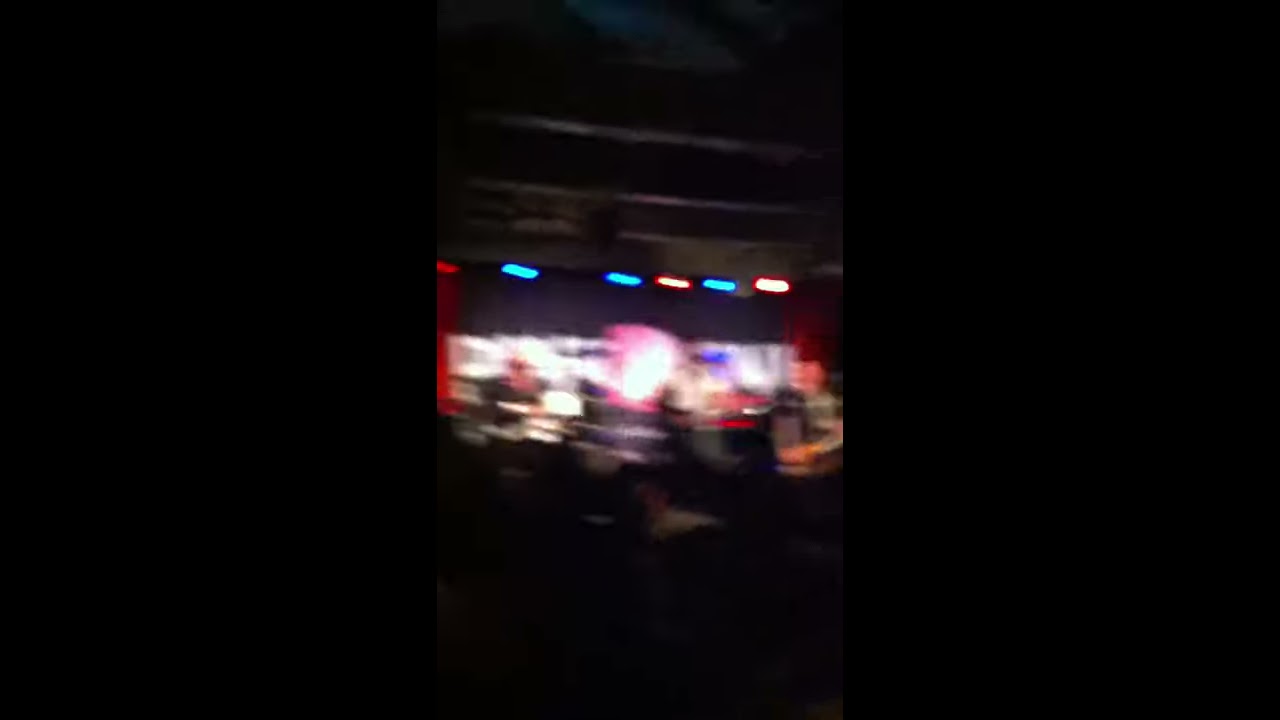The photograph is dark and very blurry, taken in portrait orientation, likely on a cell phone at night. The central focus appears to be an area with smoke or steam, illuminated by blue, red, and yellow lights positioned just above it. This illuminated section suggests it might be a stage setup, although it is difficult to determine definitively. The image features structures forming horizontal lines across the top, resembling a framework, which further hints at a stage-like environment. Below the center of the frame, somewhat obscured, are some gray shapes that could be stacked objects. Notably, there are thick black borders on both the left and right sides of the image, occupying about two-thirds of the total space. The overall image has an out-of-focus quality, with ambiguous details suggesting an unclear setting that might be either an indoor or outdoor location.